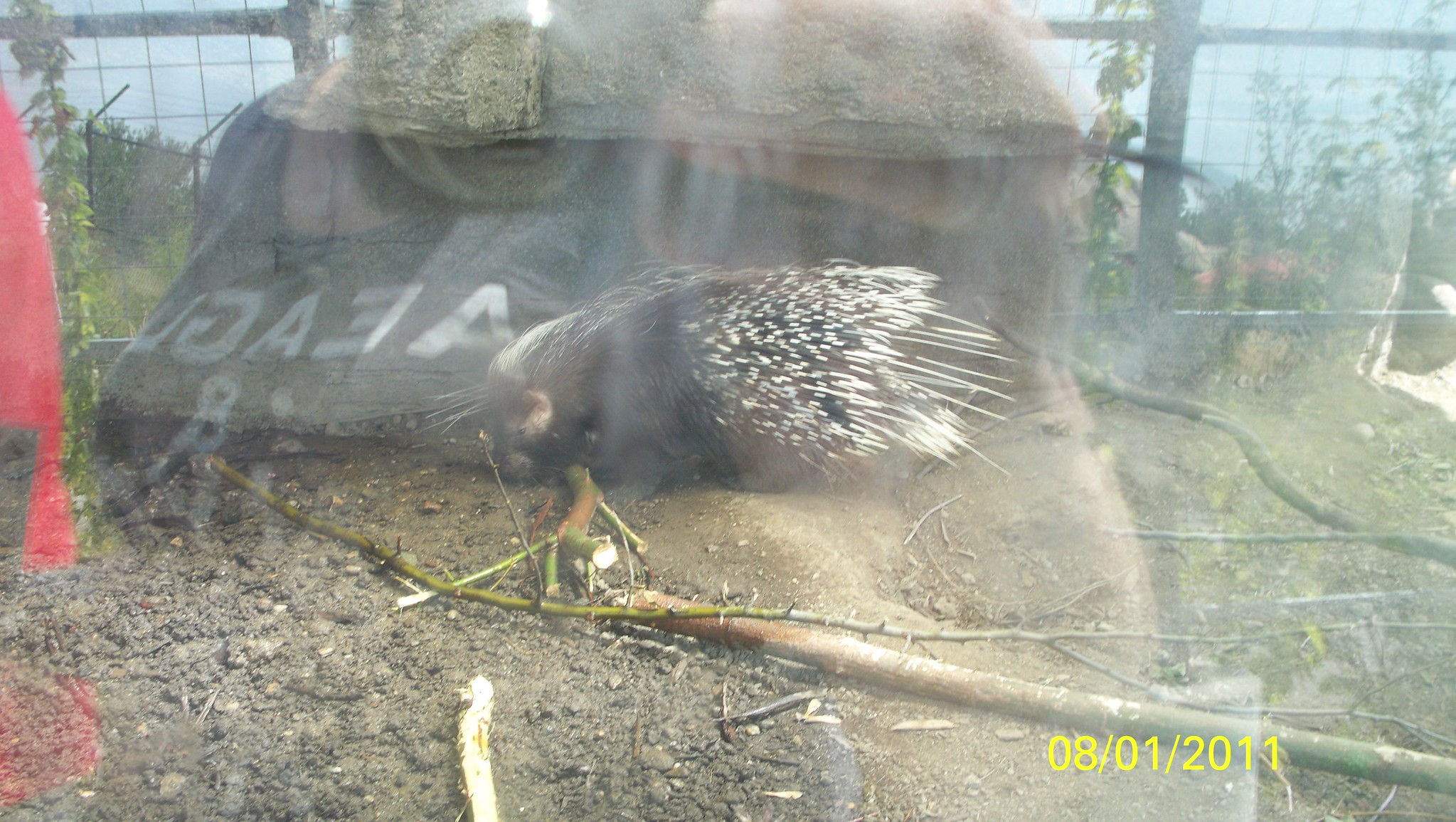The image depicts an outdoor zoo enclosure, visible through some sort of glass or transparent shield that shows noticeable reflections, though they are indistinct. The floor inside the enclosure is comprised of dry mud, devoid of grass, and is scattered with bare branches, dirt, rocks, and sticks. A medium-sized, brown porcupine can be seen in the center of the scene, facing to the left, with white coloration on its tail. To the right, there is a patch of grass, behind which a metal fence is visible, continuing toward the top left and top right corners of the image, where patches of blue sky can also be seen. Reflections on the glass show hints of the photographer and other people passing by. A yellow date stamp in the bottom right corner marks the image as taken on 08-01-2011.